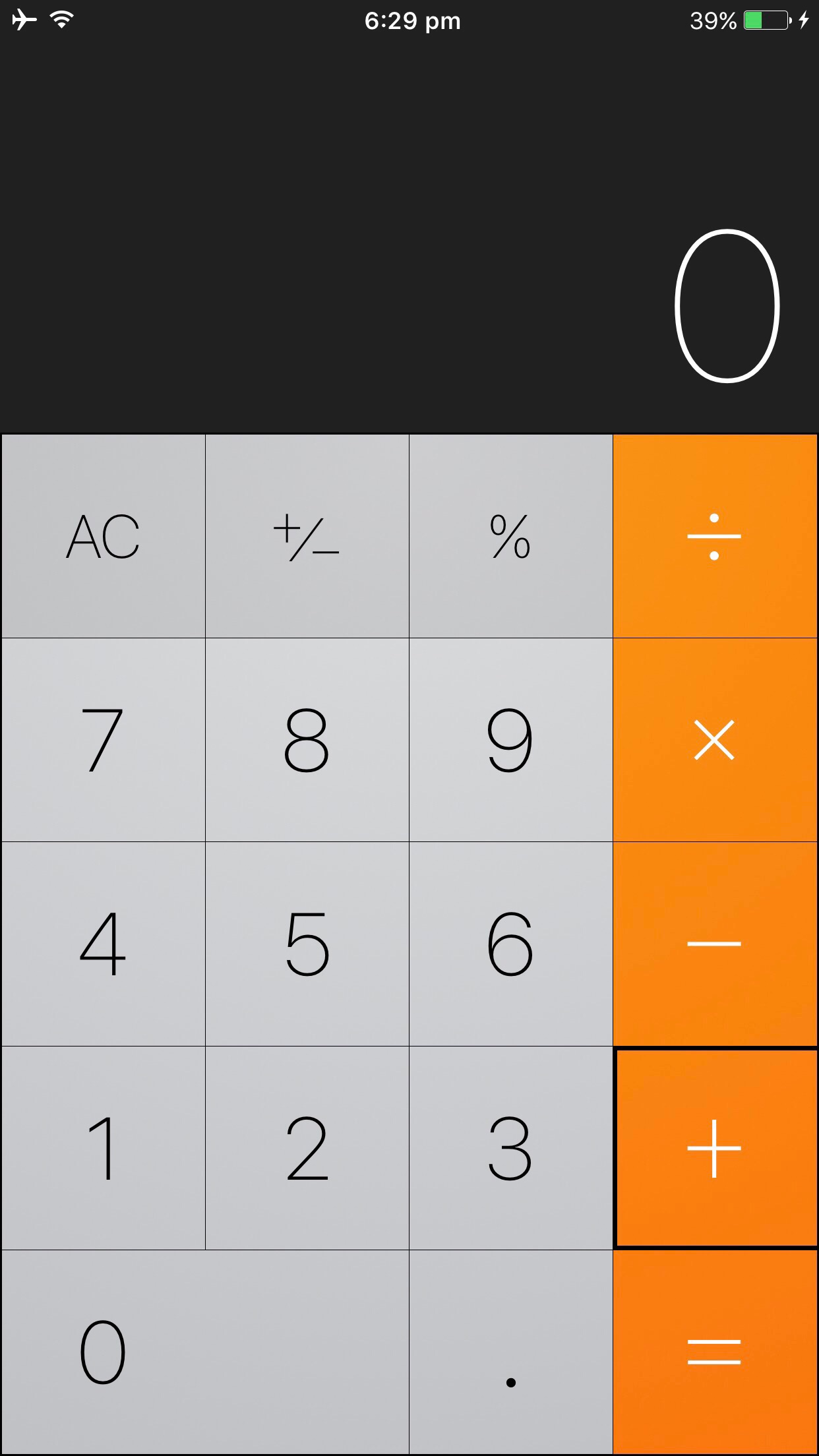The image features the calculation screen of an iPhone, clearly identified by its portrait orientation. The iPhone displays a battery life of 39% and the current time of 6:29 p.m. at the top of the screen. The device is set to airplane mode, which is indicated by the corresponding icon. Despite being on airplane mode, the phone shows good internet connectivity.

On the calculator screen, the main display area at the top shows the number zero against a black background. Below this main display are various calculator function buttons. The top row consists of "AC" (all clear), "±" (change sign), "%" (percentage), and "÷" (division). The subsequent rows display the numbers in a 3x3 grid: "7", "8", "9" with a "×" (multiplication) button underneath the division; "4", "5", "6" with a "−" (subtraction) button underneath the multiplication; "1", "2", "3" with a "+" (addition) button beneath the subtraction. At the bottom, the row features "0", a space, a decimal point ".", and an "=" (equals) button.

All operational buttons along the right-hand side—division, multiplication, subtraction, addition, and equals—are highlighted in orange, creating a vertical strip of orange-colored keys. The calculator displays no input other than the initial zero in the main display area, ready to perform calculations once a number is entered.